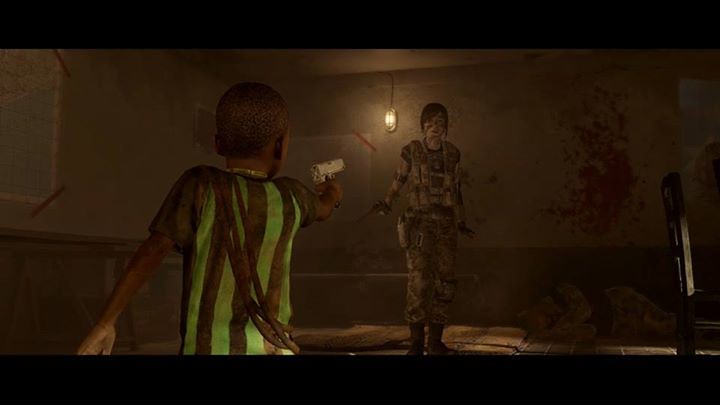This image appears to be a screenshot from an animated movie or video game, resembling titles like "The Last of Us" series. The scene is framed with black bars at the top and bottom, typical of widescreen formatting. The setting is a dismal, run-down room with industrial elements, featuring dingy cement or brick walls, and grimy, stained wallpaper.

In the center of the scene, a thin black child with very short curly black hair stands, holding a small silver gun pointed at a young Caucasian woman who looks to be in her 20s. The child, seen from behind, wears a vertically striped shirt in shades of black, green, and brown.

The young woman, who has brown hair, is clad in a military-style outfit featuring camouflaged fatigues, gloves, and black boots, with a gun holstered at her side. Her hands are raised to indicate she won’t move. Her face appears to have paint or dirt on it.

Behind the woman and to her right, there is a large red blood splatter on the wall, with a figure lying right below it who appears to be either dead or sleeping, with hands folded beneath the head. An industrial yellow light with a silver box surrounds it and is positioned on the back wall. A wooden chair sits on the right side, while a small thin mat lies on the floor. To the left, a creamy white map with a bit of blue, taped at the corners with black tape, is affixed to the wall.